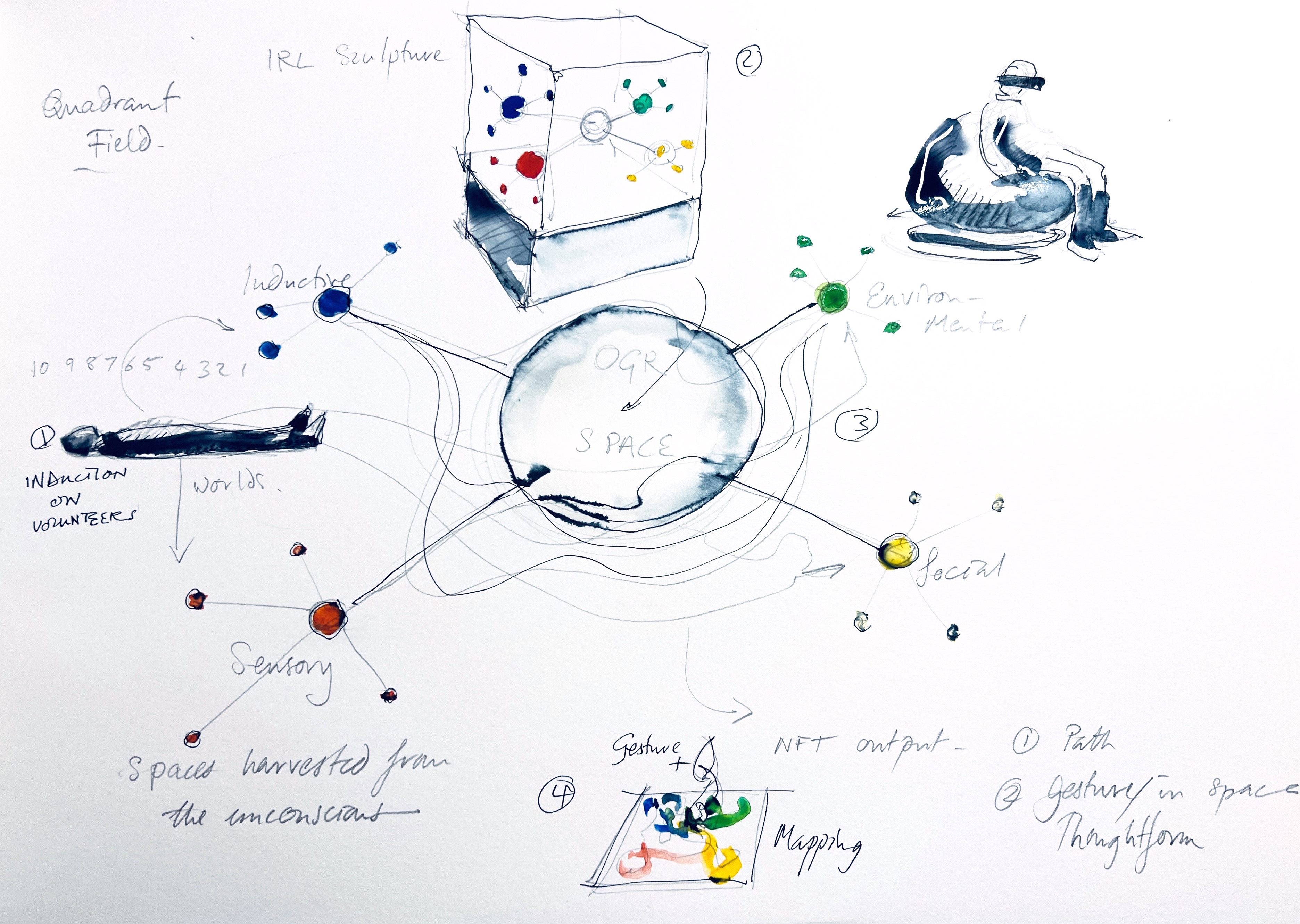The image depicts a detailed hand-drawn illustration, presumably a mix of notes from a science class. The illustration is on a blank white piece of paper, utilizing watercolor paints and pencil annotations. Central to the composition is a large pen-outlined sphere labeled "OGR space," adorned with blue watercolor stains around its edges. From this central sphere, several lines radiate outward, each connecting to smaller colored spheres with specific labels:

- To the top right, an arrow points to a green orb labeled "environmental," accompanied by three upward lines leading to smaller green circles and one line extending to the bottom right, culminating in another small green circle. Below this, a circled number "3" is present.
  
- To the bottom right, an arrow directs to a smaller yellow sphere labeled "social." This yellow sphere has four lines connecting it to four smaller white circles.
  
- To the left, an arrow points to an orange-red sphere labeled "sensory," with four lines extending to four smaller red-orange circles.
  
- Near the 10 o'clock position, a horizontal image of a body is drawn in pen, with a circled number "1" beside it and text stating "induction on volunteers" and "worlds." An arrow leads from this body image to one of the smaller red spheres. Numbers in descending order from 10 to 1, linked by an arrow, lead to a smaller blue sphere labeled "inductive," which branches out to three smaller blue circles.

At the bottom of the page, the text "space is harvested from the unconscious" is written. To the right of this, a circled number "4" is paired with the text "gesture plus," accompanied by a square featuring red, yellow, green, and blue squiggles, and the word "mapping." "NFT output" is mentioned above this section. 

Further annotations include a circled number "1" with the label "path," and below it, a circled number "2" with the text "gesture in space thought form."

Additionally, at the top right of the page, there is a watercolor illustration with blue smudges, depicting a person sitting on a beanbag chair, equipped with a device around their head, likely a VR headset. 

The title "quadrant field" is inscribed at the top of the image, indicating a systematic breakdown of complex information, possibly from a scientific or philosophical lecture.